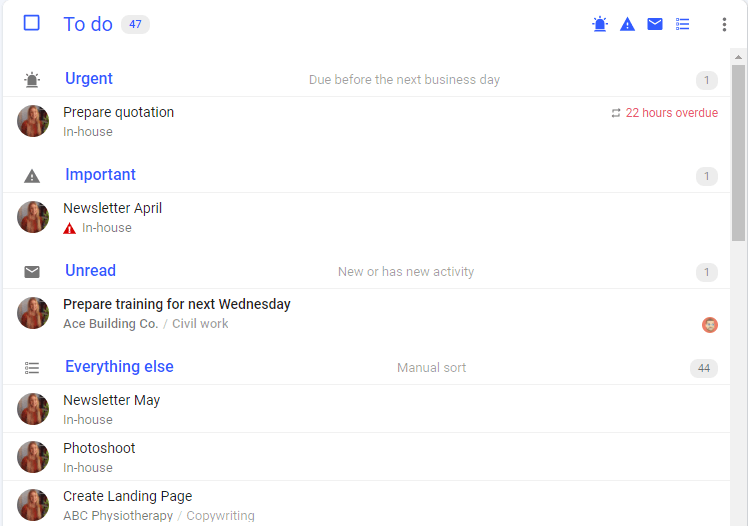A detailed screenshot with a white background showcases a blue square and a gray oval featuring the number 47. Positioned on the far right are three vertical dots, denoting additional options. The screenshot highlights an urgent task due before the next business day, marked by a red triangle with an exclamation point and the phrase "22 hours overdue." This urgent item is accompanied by a circled number 1.

The image also contains a profile picture of a lady, indicating the person responsible or involved in the task. Another profile picture, styled as a cartoon of a man, appears further down in the screenshot.

The content includes:
- "Newsletter April", signifying an upcoming or recent update.
- An envelope icon with the label "Unread", indicating new activity, again with a circled number 1.
- A task description "Prepare quotation in-house", suggesting specific preparations are needed.
- A separate task "Prepare training for next Wednesday".
- Information linked to "Ace Building Company Seal" and "Civil Work", implying the tasks are related to these projects.

Additionally, a circled number 44 is visible, which likely signifies the count of items in a category marked for manual sorting. The overall theme and structure use blue tones, giving a cohesive visual style.